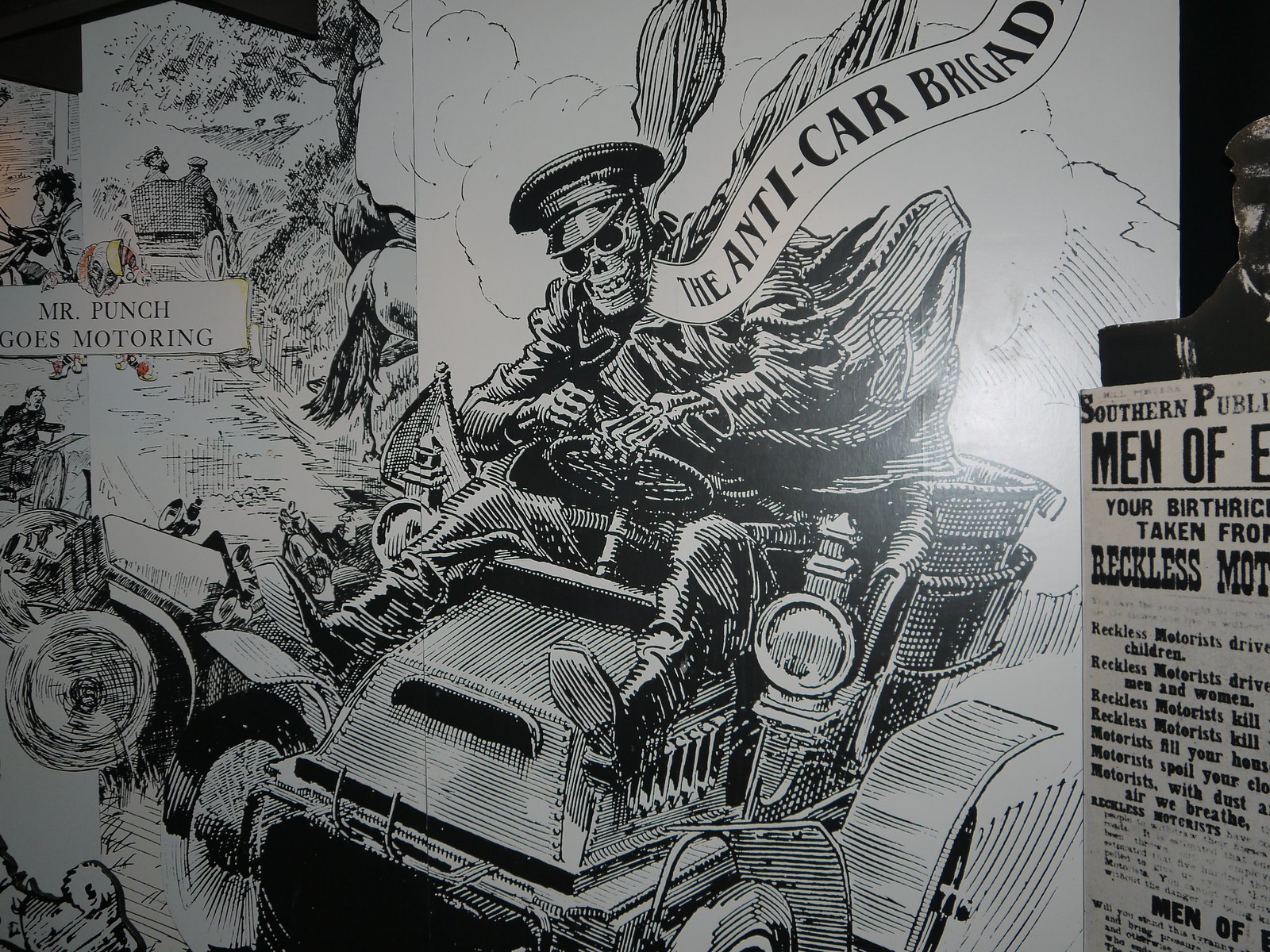This is a detailed cartoon illustration, prominently featuring a skeleton dressed in a black jacket, admiral's cap, and glasses, driving an old-fashioned car reminiscent of a 1920 Model T. The skeleton's hands protrude from the sleeves of his jacket, and a flowing black cape billows behind him. A banner emanates from the skeleton’s mouth, reading "The Anti-Car Brigade." His legs are stretched forward over the front of the car, which prominently displays large headlights.

To the upper left of the skeleton, a smaller inset sketch depicts a couple in a horse-drawn buggy with the caption "Mr. Punch Goes Motoring," accompanied by a clown-like face, alluding to the famous puppet character Mr. Punch. 

On the right side of the image, a partially visible, distressed sign warns against the dangers of reckless motoring. Despite some text being cut off, phrases like “Southern public men,” “your birthright taken from you because of reckless motoring,” and other warnings about the harmful effects of motorists are discernible. This adds to the anti-gas motor car theme of the drawing.